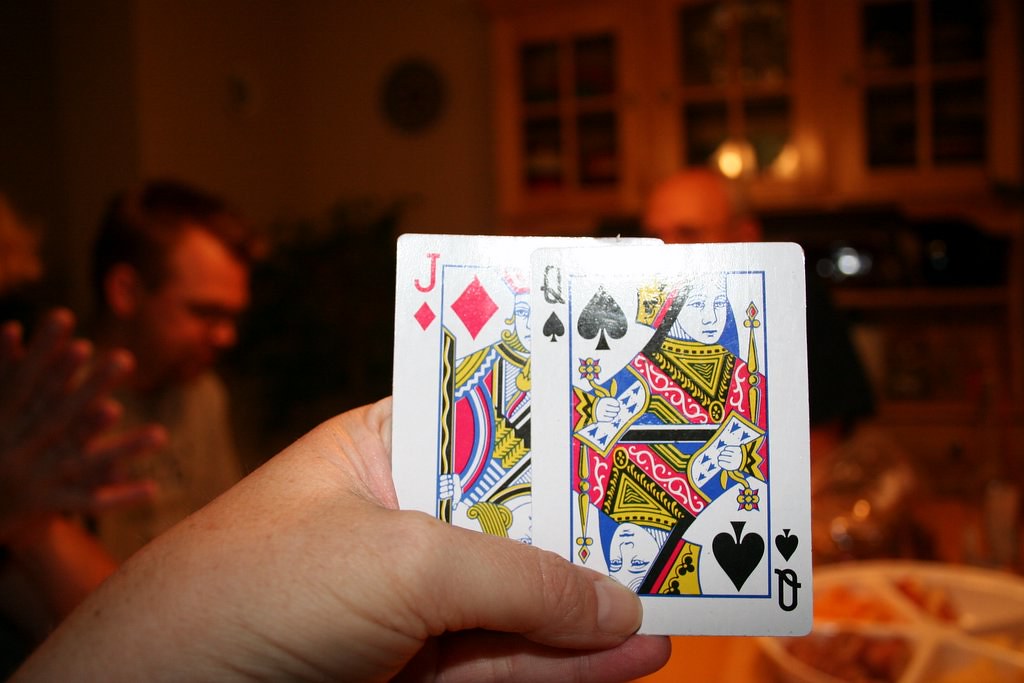In the image, a close-up shot captures a hand holding two playing cards – a joker of diamonds and a queen of spades – positioned to conceal their values from the other players at the table. The background is dimly lit, creating an intimate atmosphere. To the left, the clasped fingers of one person are visible, and next to them, a side profile of a man. Across the table, a bald man in a black shirt appears, although his face is obscured by the hand holding the cards. A dish of snacks is also placed on the table, adding to the cozy, communal setting of the card game.